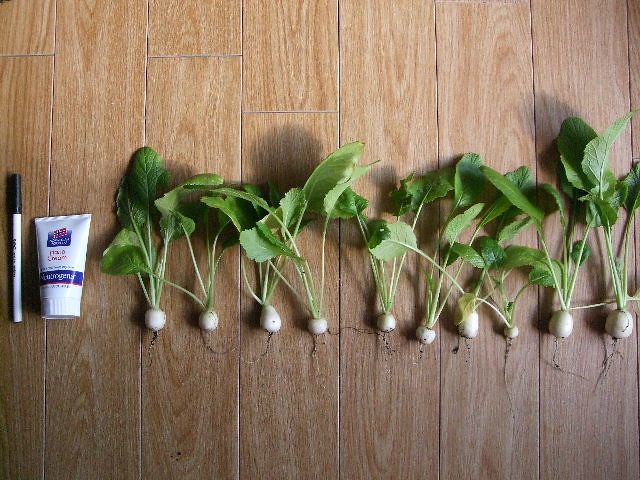This image features ten radish plants neatly arranged in a row on a brown hardwood or faux hardwood floor. To the left of the radishes, a white pen with a black top and a small bottle of Neutrogena hand cream are positioned, likely to provide scale. The hand cream bottle is white with a blue line and "Neutrogena" in white, with "hand cream" written above it in red. The radishes themselves have long green stems and leaves, with white bulbs and visible roots, indicating they have not yet turned red. Everything is centered in the middle of the picture, creating a balanced composition.